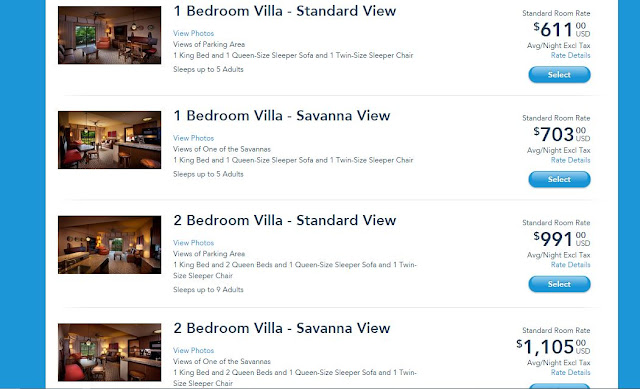The image appears to be a screenshot from a hotel booking website, displaying various accommodation options and their corresponding prices. The layout features a prominent blue bar on the left and smaller vertical blue bars on the right side of each section. Four different room options are listed, each featuring a small, somewhat dark photo on the left that is difficult to discern.

1. **One-Bedroom Villa, Standard View:**
   - **Price:** $611 USD per night, excluding taxes.
   - **Room Description:** 
     - Views of the parking area.
     - One king bed, one queen-size sleeper sofa, and one twin-size sleeper chair.
     - Accommodates up to five adults.
   - **Additional Options:** View photos.
   - **Select Button:** Not fully visible in the screenshot.

2. **One-Bedroom Villa, Savannah View:**
   - **Price:** $703 USD per night, excluding taxes.
   - **Room Description:**
     - Views of one of the savannas.
     - One king bed, one queen-size sleeper sofa, and one twin-size sleeper chair.
     - Accommodates up to five adults.
   - **Additional Options:** View photos.
   - **Select Button:** Not fully visible in the screenshot.

3. **Two-Bedroom Villa, Standard View:**
   - **Price:** $991 USD per night, excluding taxes.
   - **Room Description:**
     - Views of the parking area.
     - One king bed, two queen beds, one queen-size sleeper sofa, and one twin-size sleeper chair.
     - Accommodates up to nine adults.
   - **Additional Options:** View photos.
   - **Select Button:** Cut off in the screenshot.

4. **Two-Bedroom Villa, Savannah View:**
   - **Price:** $1,105 USD per night, excluding taxes.
   - **Room Description:**
     - Views of one of the savannas.
     - One king bed, two queen beds, one queen-size sleeper sofa, and one twin-size sleeper chair.
     - Further details about bed arrangements and capacity cut off in the screenshot.
   - **Additional Options:** View photos.
   - **Select Button:** Cut off in the screenshot.

Each room listing includes a "View photos" link in blue font for further visual details, although the sample photos provided in the screenshot are small and lack discernible details. The "Select" button for each room option is partially obscured or cut off in the image.